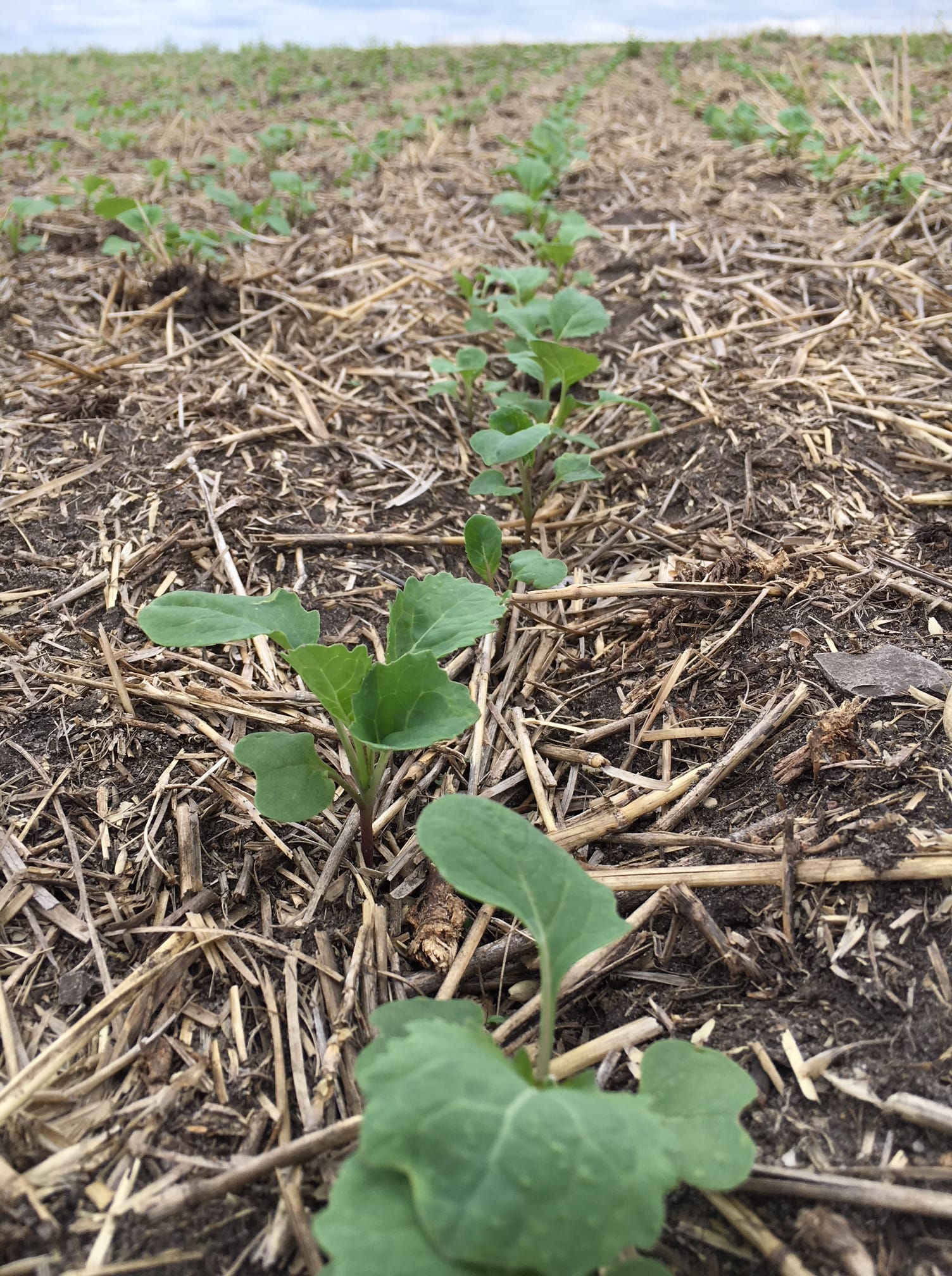This daytime outdoor photograph depicts a flat agricultural field stretching towards the horizon, captured from a low angle. A strip of blue sky with white clouds decorates the upper left and right corners of the rectangular image, signaling a clear day. Below, the field is rich with dark brown, slightly damp soil, marked by divots and lined with small, light brown, almost yellow straw. Extending from the bottom foreground towards the back lie numerous rows—up to about 50—of young green plants. Each plant emerges from a reddish-toned base, transitioning into light green stems that branch out into elliptical, darker green leaves with lighter veins. These budding sprouts appear like they could eventually grow into vegetables. The intricate details of the early-stage crops, the textured soil, and the structured rows convey a thriving agricultural setting.